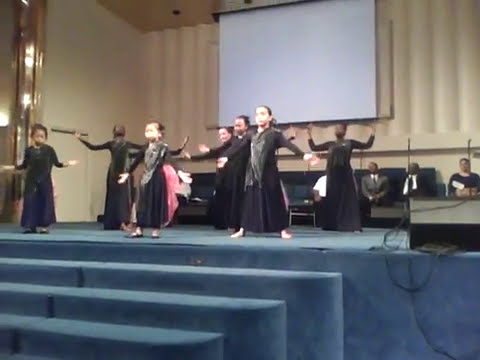In this image, a group of seven young female dancers, mostly teenagers and children, perform on a large auditorium stage. The stage is notably covered in light blue velvety material, and it includes a set of blue velvet-covered stairs at the front. The dancers, all dressed in black dresses with long scarves, exhibit movements with their hands and arms extended in various positions; some dancers have their hands raised high while others have them lowered towards the floor. A mix of barefoot and ballerina shoe-clad feet are visible.

Behind the dancers, the auditorium is characterized by a beige backdrop featuring a large, empty white projection screen and a columned, tiled wall that adds texture to the background. The spaciousness of the stage is evident, suggesting ample room for the performance.

In the background, a seated audience of adults, including men in suit shirts and at least one woman, attentively watch the performance. The blue seating area contrasts with the stage and creates a distinct separation between the performers and the spectators. Additionally, an emergency exit door is located in the corner of the stage area, hinting at the structured layout typical of such venues.